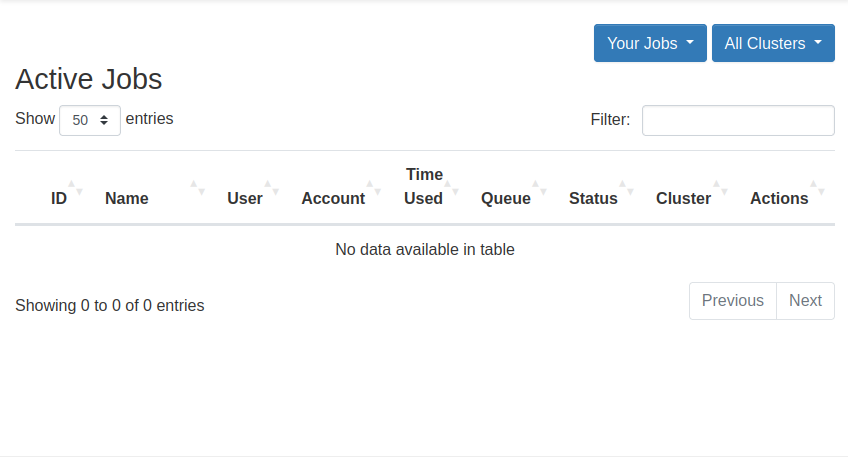A detailed screenshot of a computer interface, likely related to server administration, is displayed. The image, captured on a desktop or laptop, shows an empty job queue within a software panel. At the top left corner, a header labeled "Active Jobs" is visible, accompanied by a drop-down menu allowing the user to "Show 50 entries". On the top right, two blue buttons are labeled "Your Jobs" and "All Clusters," suggesting toggles for filtering job views. Below this, a search box is present for filtering entries by specific criteria.

The main table beneath the search box is organized into several columns: ID, Name, User, Account, Time Used, Queue, Status, Cluster, and Actions. Despite the organizational structure, the message "No data available in table" indicates the absence of any job entries. Below the table, a footer notes "Showing 0 to 0 of 0 entries." Additionally, navigation buttons labeled "Previous" and "Next" are present but disabled, confirming the lack of data to paginate through.

The layout appears to be in a widescreen format, slightly cropped and zoomed in from a larger original image, reflecting its focus on this specific interface section. Without additional context, the primary function of this interface remains speculative, though it strongly resembles a job queue management system used in server administration.